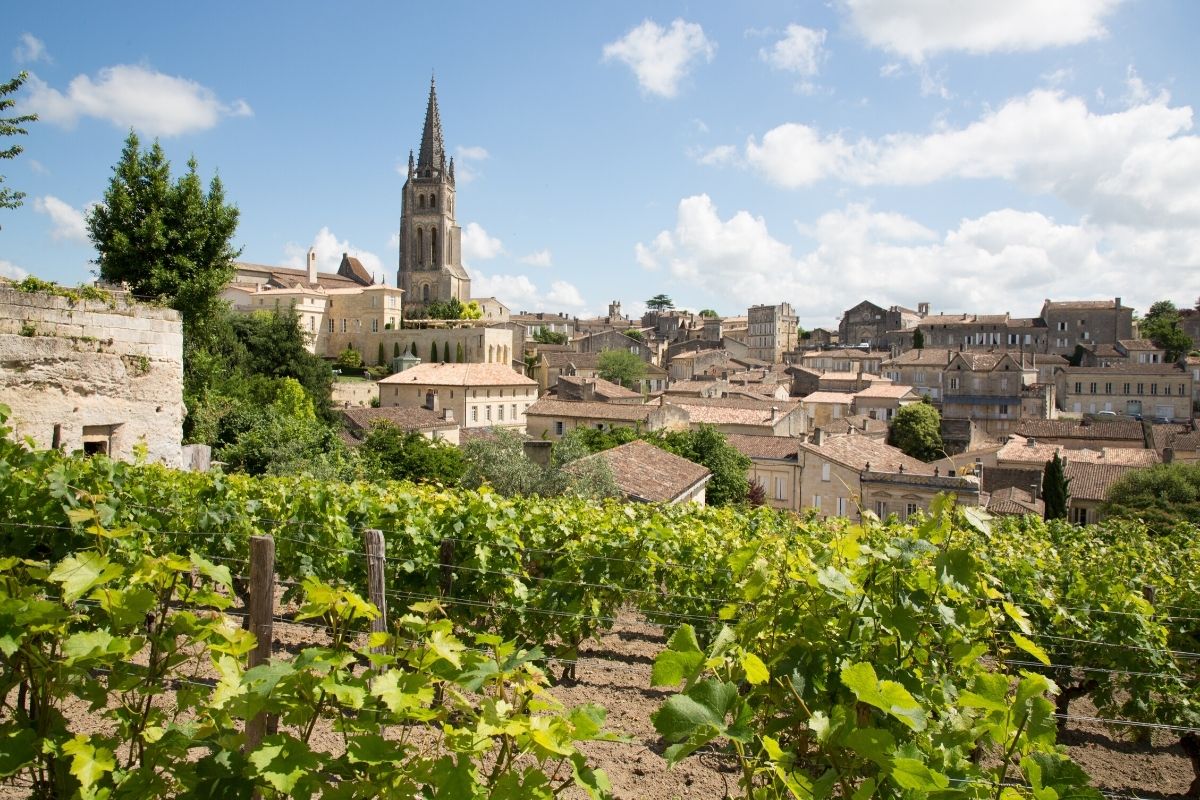The image portrays a picturesque scene of what appears to be a Greek or European city bathed in bright sunlight, suggesting a warm and cheerful day. In the forefront, a lush vineyard with tall, sunlit plants is crisscrossed by supporting wires and a fence, hinting at early afternoon with distinct, hard shadows. A small, old brick structure covered in moss stands to the left, adding a touch of antiquity. Beyond the vineyard, the city unfolds, characterized by close-set buildings in varying heights but predominantly in shades of tan, brown, and cream. Off in the distance to the left rises a tall spire, likely a church, distinguishable by its gray top. The sky above is a mix of pale blue with wispy clouds concentrated in the upper right, contributing to a slightly hazy yet partly cloudy atmosphere. The scene gives a sense of warmth, history, and communal life, portraying a densely built, non-modern cityscape with significant architectural variety.